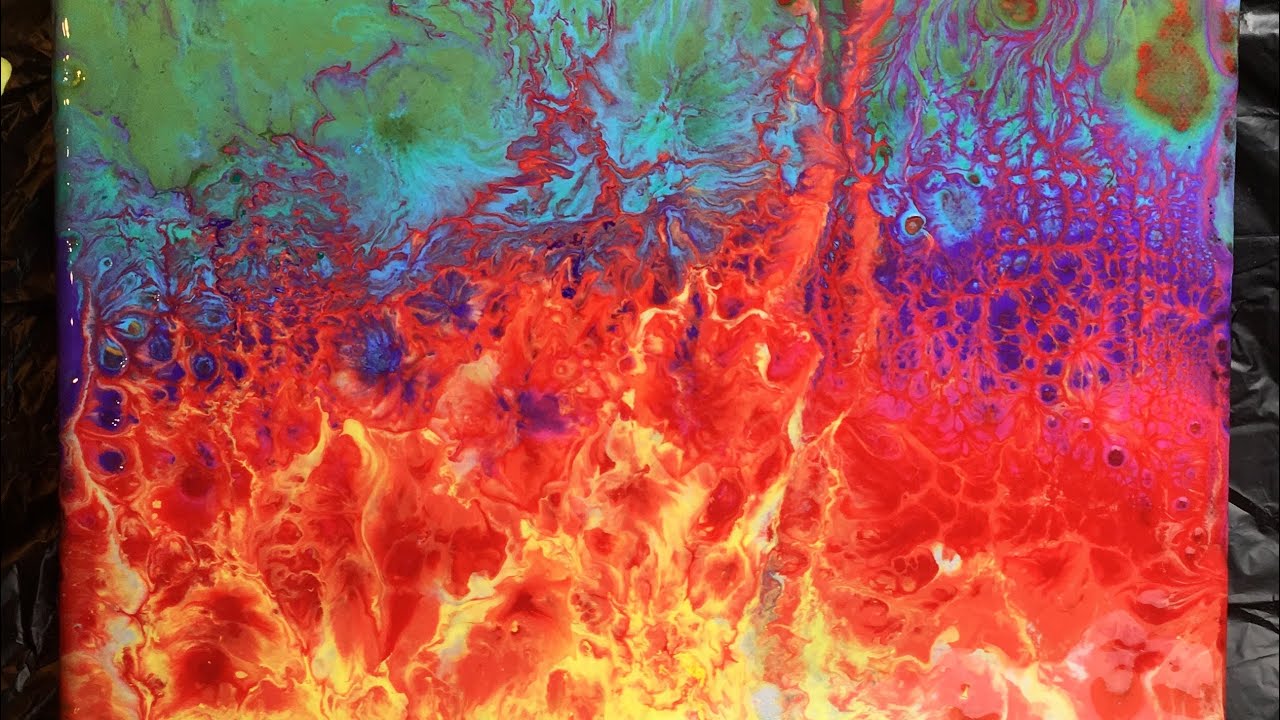This image is a vibrant, psychedelic painting resembling a vivid, explosive fire. At the bottom, the painting starts with bright yellow and orange, almost white-hot flames that gradually transition into a mix of red, reminiscent of an intense explosion. As the flames rise, they morph into jagged, branching forms rather than smooth, rounded bubbles, stretching upwards into a cascade of colors including purple, blue, and green. The artwork evokes the chaotic beauty of flames merging with an abstract, colorful background. The image suggests an oil spill or a hazy, infrared-like effect, enhanced by its glossy, fluid appearance. Set against a dimly lit studio, possibly with a visible tarp on the floor, the contrasting background emphasizes the radiant, fiery spectacle in the foreground.